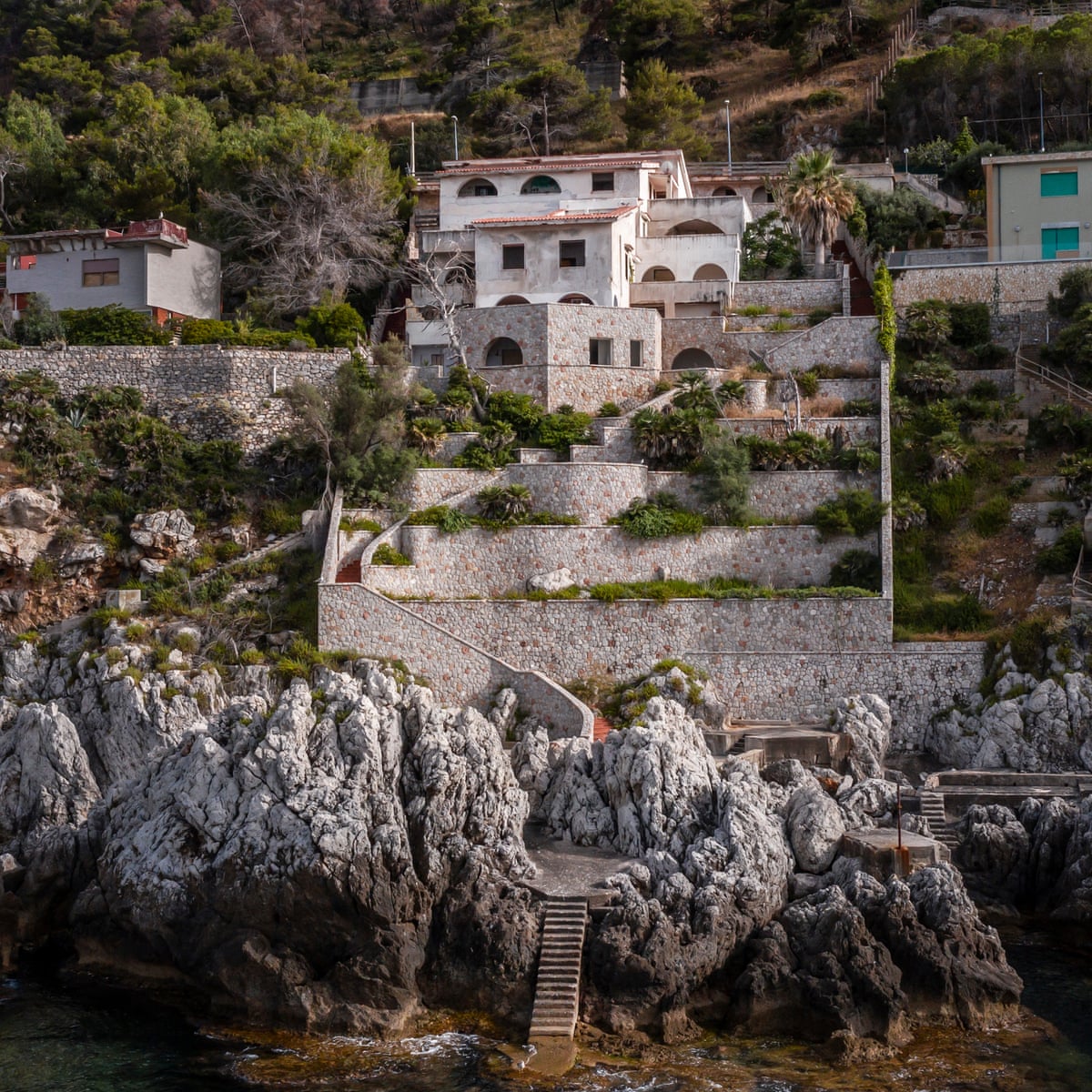The photograph captures a daytime, full-color image of a cliffside adorned with buildings and intricate stonework. At the base, you see a craggy, rocky area with gray rocks that transition to brown as they approach the water, likely indicating the waterline's effect. Central to the image is a set of steps or ladders that ascend from the water's edge through the rocky terrain, leading to a terraced hillside.

On the cliff, various structures are integrated into the landscape. Dominating the scene is a white hacienda-style mansion with a pinkish roof, situated several levels up the cliff. To the left of this central mansion is another white building with a red roof, and to the right, a white building featuring turquoise windows or doors. Each building is nestled among multiple stone walls and gates, which are predominantly white but interspersed with other colors.

The terraced ascent includes a combination of steps and fortified walls, climbing from the water's edge upward, with green shrubs and vines decorating the lower layers. As the elevation increases, more green trees and bushes become visible, blending with the stone structures. The topmost portions of the cliff feature additional greenery, suggesting a gradual transition from built environment to natural mountain landscape.